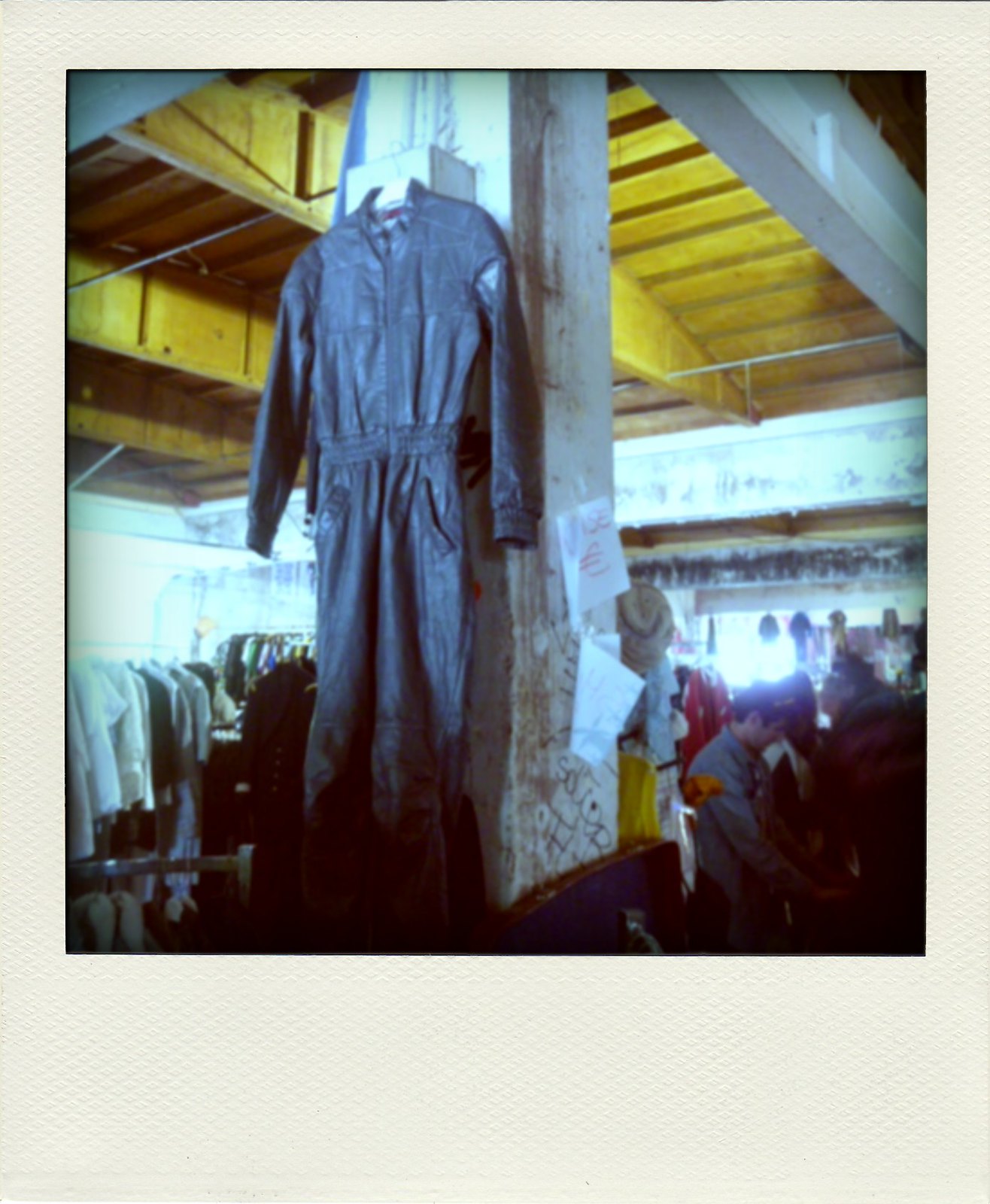The photograph depicts the interior of a clothing store, possibly an international or thrift shop, characterized by its industrial and somewhat eclectic aesthetic. The focal point of the image is a gray leather or vinyl jumpsuit that hangs prominently from a white hanger on a central cement column adorned with graffiti and various flyers. This one-piece jumpsuit, reminiscent of attire worn by mechanics, motorcycle racers, or pilots, features multiple pockets on the lower half. The store has a mix of modern and rustic elements, with wooden rafters and a ceiling tinged in light brown hues. Yellow lighting casts a warm glow throughout the space, accentuated by natural light filtering in. Clothing racks filled with various garments populate the lower left side of the image, while several shoppers, including a man, are seen perusing items on the right. The upper portion of the photograph showcases the shop's structural details, including wooden features, some painted white, which hint at an international setting, possibly Asian, suggested by the foreign script visible on a back wall.